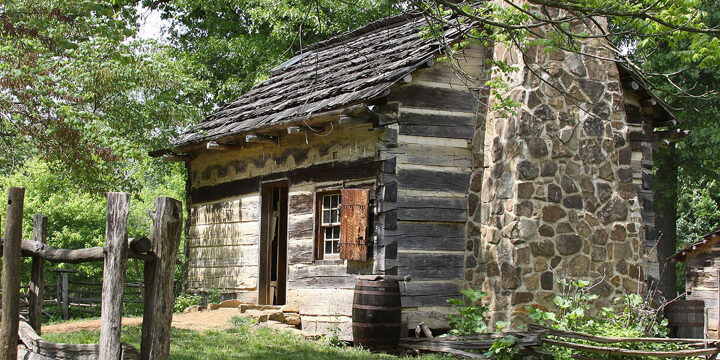This image captures a rustic wooden cabin situated in a serene forest, surrounded by dense trees with green foliage. The cabin is constructed from weathered grey wooden logs and features a pitched, triangular roof. Prominently displayed on the front wall is a single window to the right and a door positioned centrally. 

Adjacent to the cabin, a cylindrical wooden water barrel rests on the ground, while a stone chimney is attached to the side. A wooden log fence extends from the bottom left, partially encircling the cabin. The scene is set on a sunny day, with colors that include various shades of brown, grey, green, and light tan for the walkways leading up to the doorway. This idyllic snapshot evokes a peaceful, country atmosphere.